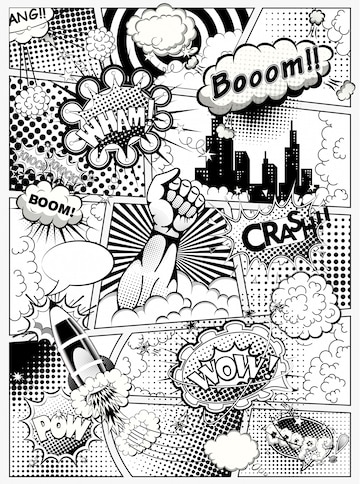This black and white image, oriented in portrait mode, captures the dynamic energy of a comic book page filled with action and chaos. The collage is segmented into seemingly random frames, each decorated with classic comic book elements. Clouds of smoke, dots, lines, and hypnotic patterns fill the background, contributing to the sense of pandemonium. Dominating the scene are multiple expressive word bubbles with exclamations such as "Boom," "Wham," "Crash," "Wow," "Pow," and "Oops." A prominently displayed muscular fist reaches skyward in the center, exuding power and anger. To the lower left, a rocket propels amidst smoke trails, adding to the frenetic activity. The collage also features a small cityscape, a knock knock joke, additional word bubbles, and various stereotypical comic book tropes, creating a visually rich and immersive experience that pays homage to vintage superhero comics.